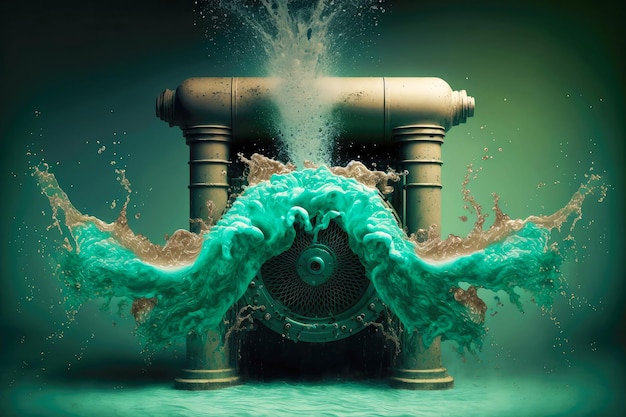The digital creation depicts an underwater scene dominated by a large, pressurized machine, appearing as a golden-colored, U-shaped object with two prominent columns on either side. Centered between these columns is a circular mechanism vigorously spinning green liquid mixed with brown dirt. This machinery seems to generate a chaotic environment underwater, with splashes and eruptions of blue water, brown liquid, and thicker greenish-blue liquid shooting out symmetrically from the front and sides. The surrounding water has a greenish hue that darkens to almost black at the top of the image, creating a rough and turbulent underwater ambience.